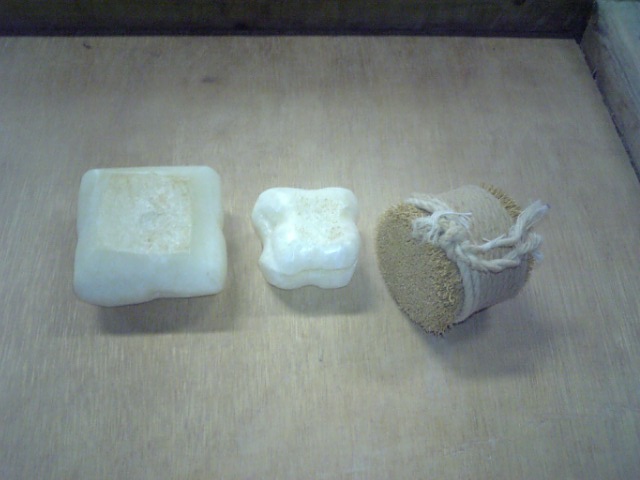The desaturated color photograph features three distinct objects aligned horizontally on an unfinished piece of plywood or possibly a grey, pale brownish surface, with a grey wall visible in the upper right corner. The image has a muted palette, consisting mainly of cream, beige, grey, and black tones.

On the far left is a white, squarish object, somewhat irregular in shape, with brownish markings on its top surface. It isn't a perfect square, as its right-hand side appears smaller than its left at the bottom.

In the center is another white object, resembling a molar tooth in shape but not an actual tooth. It features faint brown markings on its top. There appears to be a line through its middle, suggesting it could potentially open like a case.

The object on the right is cylindrical and placed diagonally. It is a small bundle of straw or grass fragments, tied together with white string, giving it a rustic appearance. The bundle is primarily a beige-brown color with lighter beige rims and a black upper edge.

These objects are meticulously arranged, providing a contrasting visual against the unfinished plywood backdrop, creating a scene of peculiar yet intriguing everyday items.